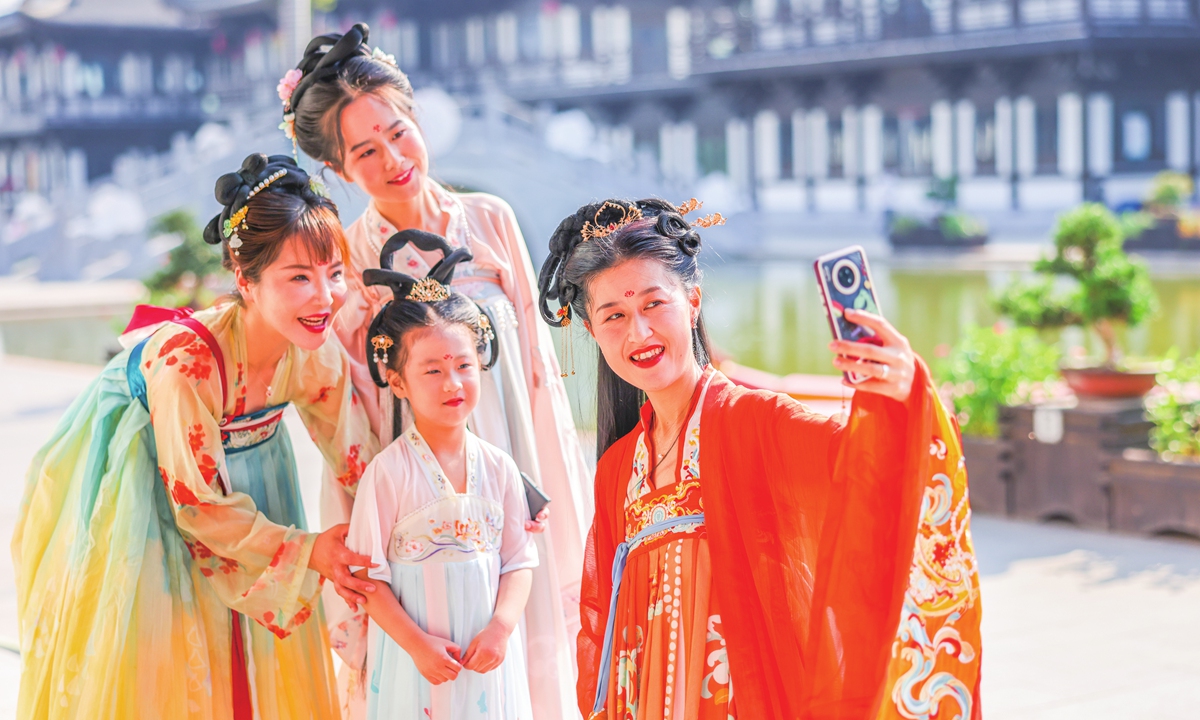In this vibrant outdoor selfie taken on a sunny day, the scene is set in a picturesque Asian city, possibly Japan or China, featuring a backdrop of blurred black-and-white buildings. A serene body of green water winds through the landscape, bordered by potted plants and bonsai trees. In the foreground, four figures are grouped closely together, smiling warmly for the camera. Three women and a little girl are dressed in intricately detailed traditional attire, showcasing the rich cultural heritage of the region. The women wear kimonos in striking red, blue and yellow, and pink hues, with their hair meticulously styled and adorned with black bows and decorative hairpieces. Each has red lipstick and a distinct red dot centered on their forehead, enhancing their classic appearance. The little girl matches their elegance in a charming light pink and blue kimono. The woman on the right, dressed in an orange-red kimono and wearing a red dot, holds up a smartphone decorated with a green cartoon dinosaur, capturing this joyful moment against the scenic cityscape.